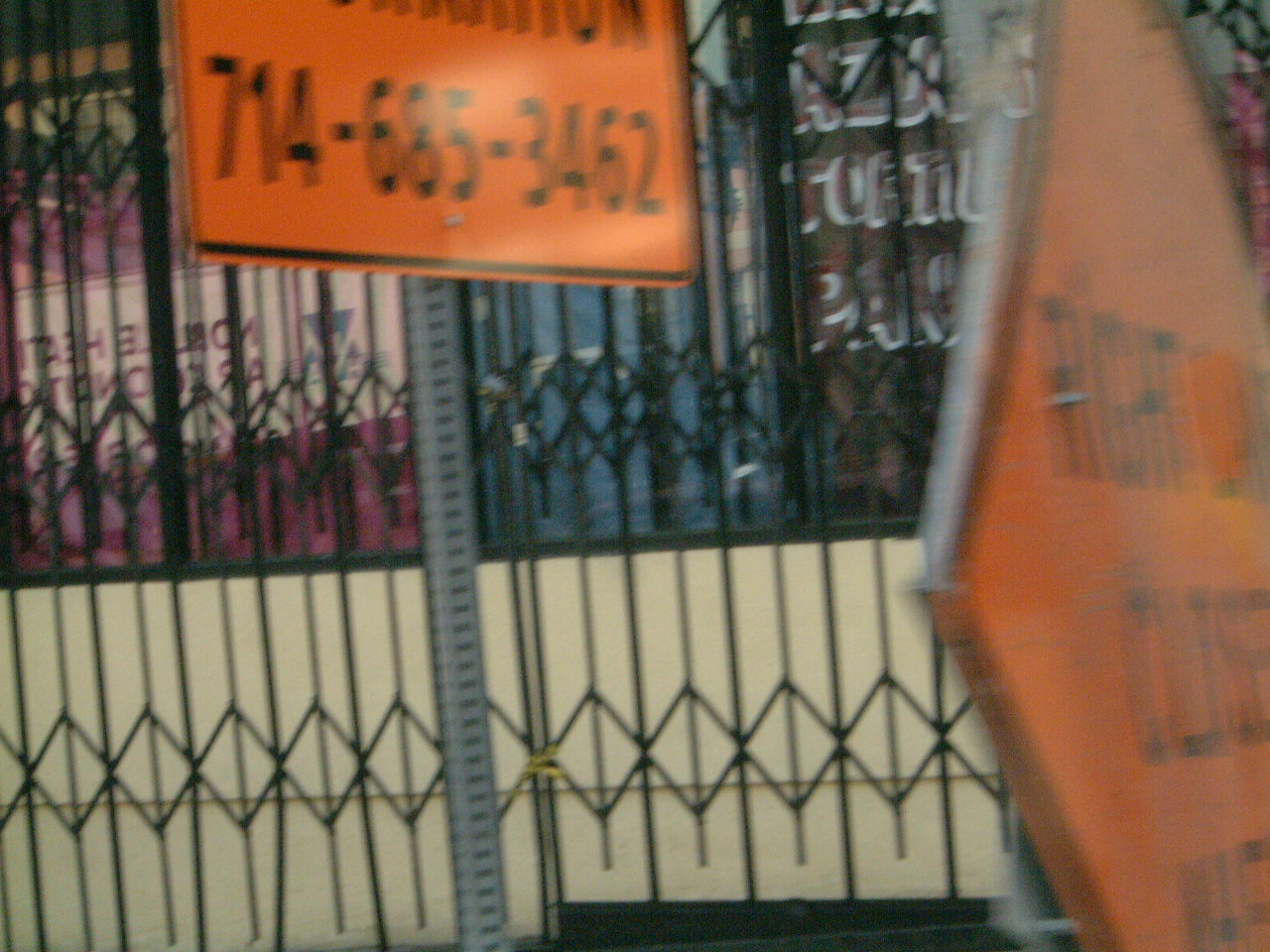This color photograph, taken outdoors, captures a pair of orange signs against a blurry, moving backdrop. On the left side, mounted on a grayish-silver metal post, is a rectangular orange sign featuring the readable phone number 714-685-3462, framed with a black rim. To the right, slightly more blurred, is a diamond-shaped orange sign with black text that appears to include the letters "R" and "CUS," though it remains largely unreadable due to the angle and focus. In the background, a black metal fence, characterized by a diamond design, secures a building with several glass windows adorned with indistinct text. The scene suggests a dynamic environment, possibly captured while the photographer was in motion, lending a sense of immediacy to the image.